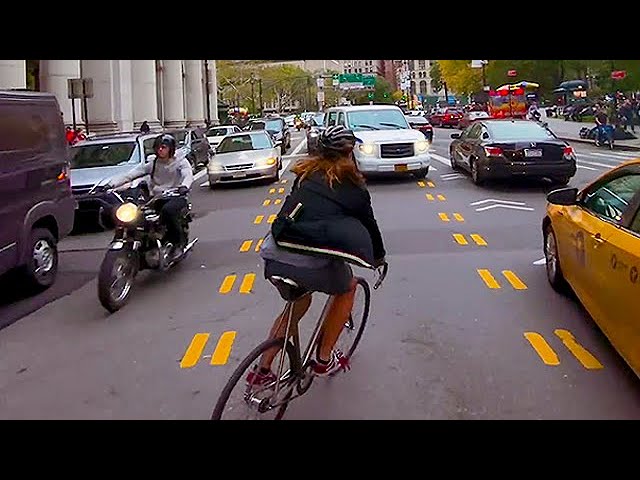The photograph depicts a bustling city street, likely captured from a video given the presence of black bars above and below the image and noticeable heavy compression. In the image, a woman in a black jacket and helmet is cycling, taking a right turn in the middle lane amidst dense traffic. To her right, a yellow taxi or car moves alongside, while to her left, a motorcyclist in grey attire and a black helmet rides in the opposite direction. The woman is observed from behind, her direction being away from the viewer. Further ahead, other vehicles contribute to the busy scene, including a white car in the middle lane, a black car in the top right corner, and a grey car to the left. The street teems with activity, including pedestrians on the sidewalk. Dominating the left side of the image is a large building with white pillars, suggestive of a library or a governmental structure, adding to the urban atmosphere and the setting's bustling energy.